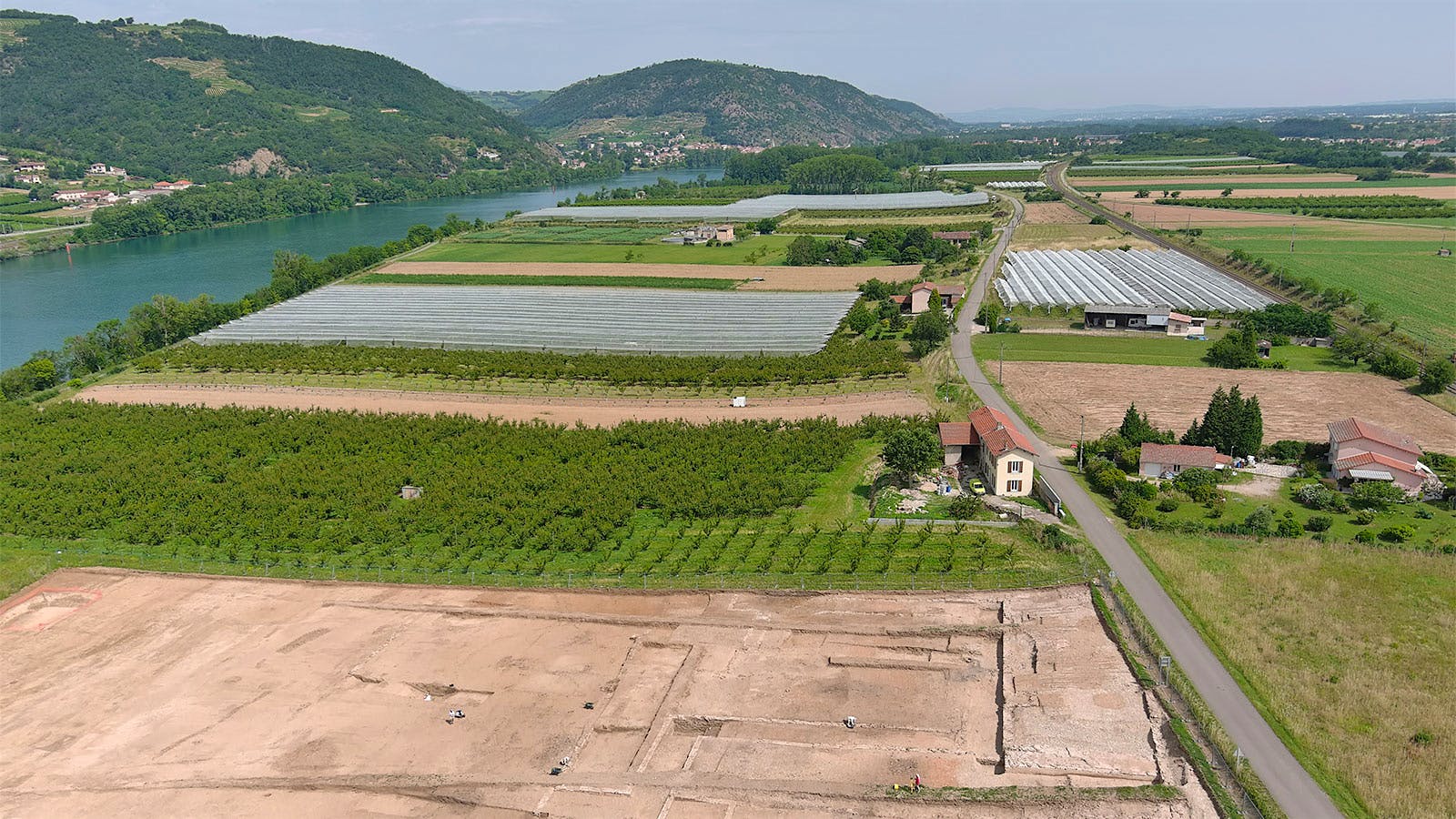This aerial photograph captures a serene rural landscape bathed in daylight. Dominated by an expansive section of water to the left, the scene showcases a blue river meandering through fields of dirt and patches of grass. In the background to the left, imposing, tree-covered mountains rise, creating a dramatic natural backdrop. To the right, sparsely scattered white houses with light red roofs dot the landscape, set far apart amidst vast tracts of open land, highlighting the area's rural and spacious character. A gray road runs through the middle of the image, connecting the fields and the houses, emphasizing the sparse yet picturesque habitation. The colors of the landscape blend harmoniously, with shades of brown and green contrasting with the blue of the river and the light blue of the sky, depicting a typical peaceful countryside scene from a height that affords a comprehensive view of the town and farm below.